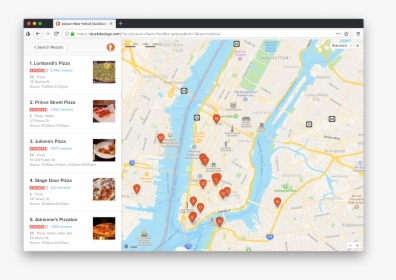In the screenshot, the background features a detailed map of a peninsula adorned with numerous red icon logos, indicating various points of interest. On the left side of the image, there is a vertical list of pizza places, although the text is somewhat small and difficult to read. 

Each listing includes a small picture of a pizza and the name of the establishment. The pizza places mentioned are Lorraine's Pizza, another place with an 'L' that is somewhat unclear, Peace Street Pizza, Place Street Pizza, Jelani's Pizza, Stage Door Pizza, and Climbers Pizzeria. The ratings for these establishments are also visible, with Stage Door Pizza and Climbers Pizzeria both having four stars. Jelani's Pizza boasts a rating of four and a half stars, as does Peace Street Pizza. Lorraine's Pizza, the first on the list, also has a four-star rating.